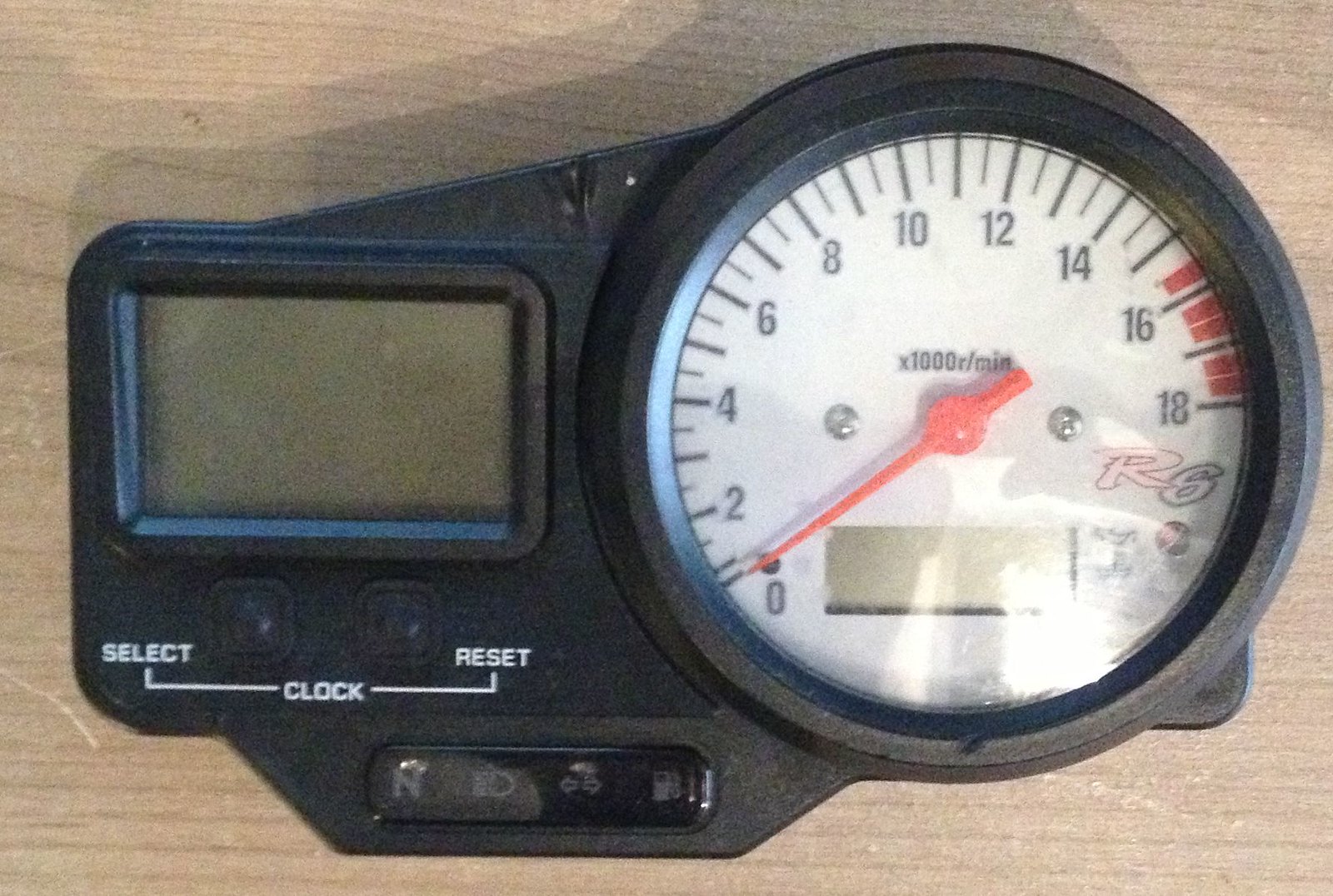This horizontally rectangular, grainy photograph captures a scene featuring a small black machine, likely a clock or similar device, placed on a table or counter with a medium-colored wooden background. The device has a white-faced clock set within a black frame. The clock's face prominently displays "X1000R / MIN" in the center, and "R6" in the lower right corner. The clock markings start at 0 on the lower left and increment by twos up to 18, labeled as 0, 2, 4, 6, 8, 10, 12, 14, 16, and 18.

Attached to the left side of the clock is a small, unlit screen. Below this screen are two black square buttons labeled "select clock" and "reset." The light source appears to be coming from the lower right, casting a shadow of the small black machine onto the wooden background in the upper left corner of the image. The overall setting suggests a blend of functionality and simplicity, with the device and its details standing out against the warm wooden backdrop.